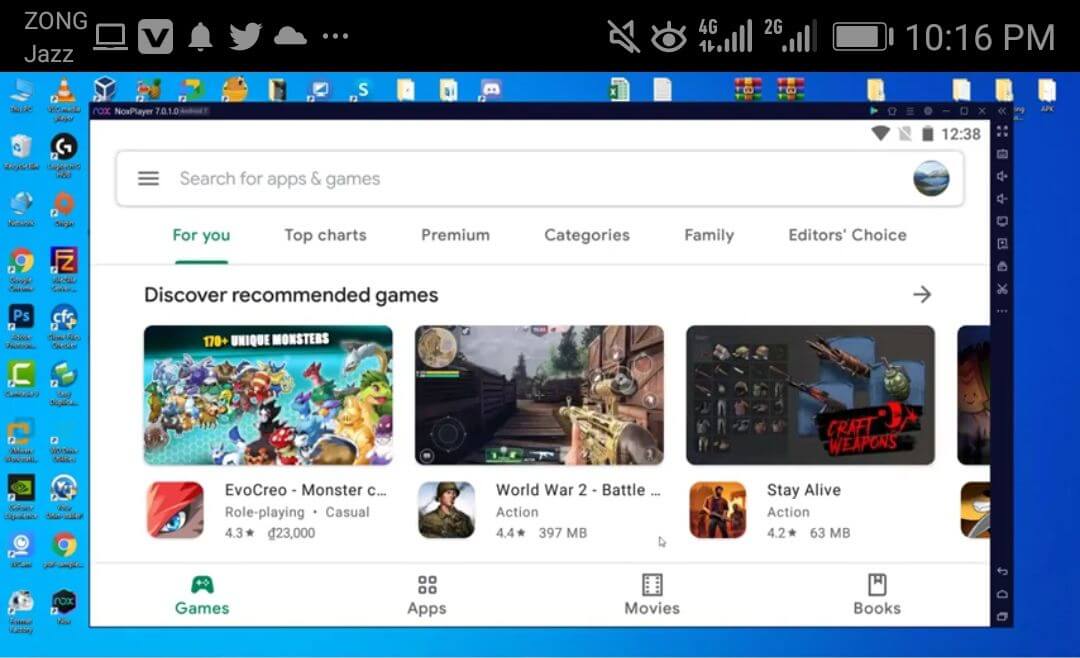The image appears to be a screenshot of a desktop interface. The top menu bar includes service providers "Zong" and "Jazz." Social media links are visible alongside indicators showing that the volume is muted and the brightness level. The 4G signal strength is full, the battery level is adequate, and the time is 10:16 AM.

The open window displays a search bar with no text entered. However, the page seems to reflect previous activity as it showcases tabs labeled "For You," "Top Charts," "Premium," "Categories," "Family," and "Editor's Choice," with the "For You" tab currently active. This tab is presenting recommended games.

Highlighted games include:
1. **EvoCreo Monster Something**: This game features a banner indicating it has 170+ unique monsters.
2. **World War II Battle**: Although the full title isn't visible, the partial name and image suggest a first-person shooter game set in a historical wartime environment, complete with guns, trees, and scattered supply crates.
3. **Stay Alive**: The caption "Craft Weapons" and background elements such as guns and building materials suggest this is another shooter game focusing on survival and crafting mechanics.

The website appears to be a platform for discovering and recommending games based on user preferences.